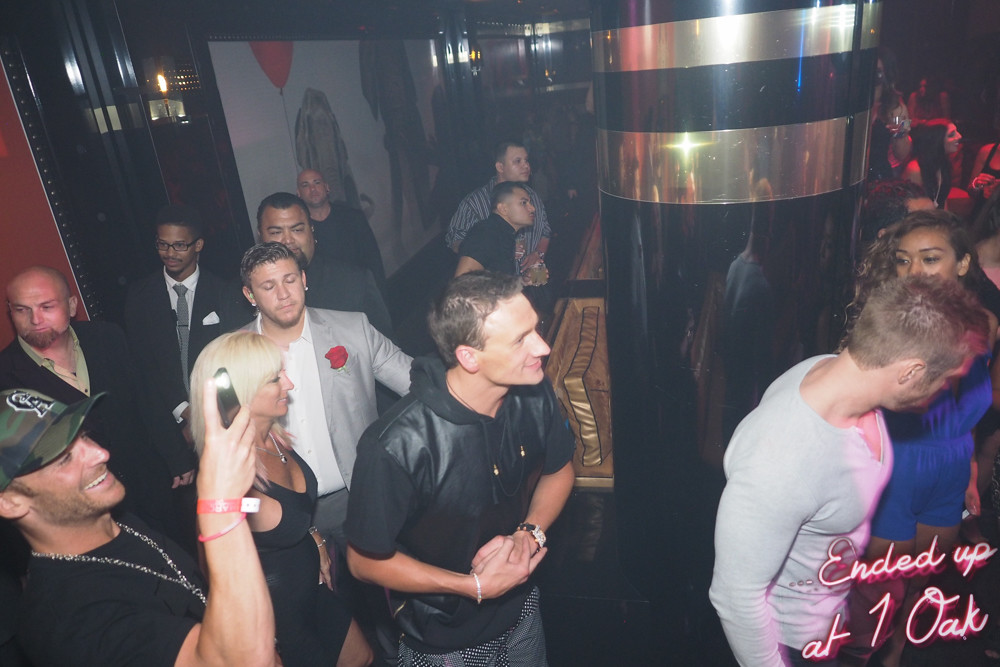The image captures a lively scene at the One Oak nightclub. Multiple people, dressed in a mix of formal suits, snazzy casual clothes, and vibrant party attire, are mingling in an ornate room adorned with shiny black doors and a combination of gray and red walls. Central to the scene is a large pillar, striking with its shiny gold and black stripes, around which people are gathering. The focal point is a man in the center wearing a shiny black leather-like shirt and fancy gray trousers, while to his right stands a man in a tight-fitting light gray shirt. Behind them, a blonde woman and another woman in a dark purple-blue dress and shorts add to the vibrant mix of party-goers. At the bottom of the image, neon pinkish-red text reads "ended up at One Oak," indicating the name of the club. Party-goers are seen dancing, taking photos, and overall enjoying the energetic atmosphere of the nightclub.